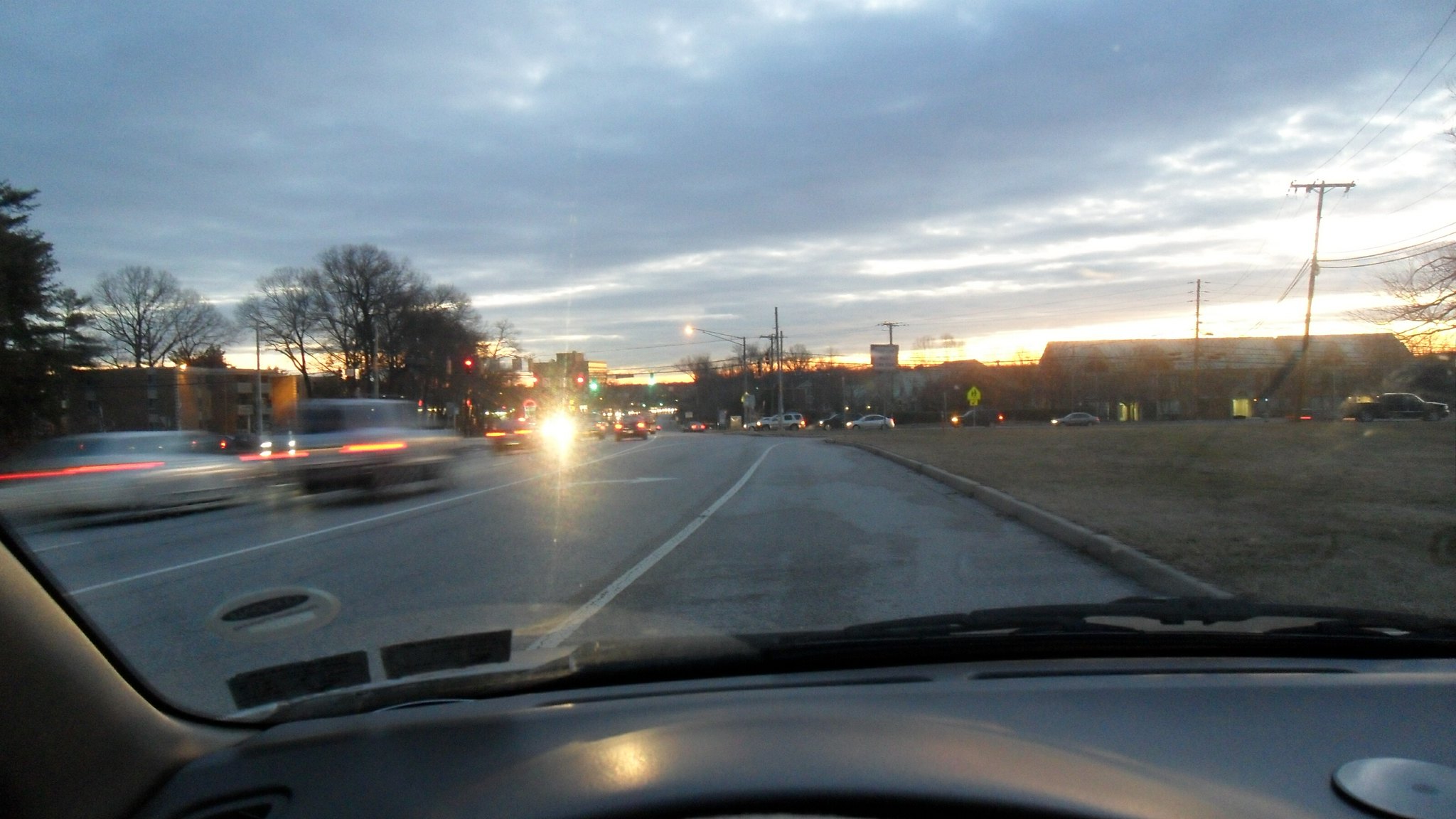This detailed photograph captures a scene from within a car that is pulled over onto the shoulder of a road, adjacent to a right turn lane. The viewpoint is from the driver's seat, looking out through the windshield where elements of the black dashboard and windshield wiper are visible. The road ahead is a four-lane street with cars moving away from the intersection under a green light, which notably casts a super bright glow. In contrast, cars heading in the opposite direction are lined up at a red light, waiting to cross the intersection. The sky is overcast with a continuous layer of clouds, signifying it is nearing dusk, adding a dim, ambient light to the scene. The surrounding environment includes a curb, a grassy area, bare trees indicating late fall, telephone poles with lines, and several buildings including a three-story apartment. The combination of blurred car movements and stationary objects adds depth to the image, highlighting the dynamic yet calm moment during sunset.